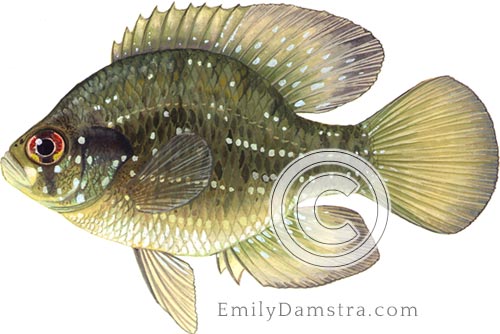This highly detailed, true-to-life painting captures a vibrant, freshwater fish, possibly a perch or juvenile bass. The fish features an intricate palette dominated by pale green and gray hues, interspersed with dark green accents. Its scales are meticulously rendered, showcasing white dots scattered across its body. The belly transitions into lighter shades of white and beige. It has a striking eye, yellow with a red ring around the black pupil, adding to its lifelike appearance. The fish boasts a prominent dorsal fin, large tail, and additional fins towards its bottom. Notably, the tail exhibits dark green tones with even darker accents. The image is set against a white background, with a noticeable copyright mark on the body. At the bottom of the painting, the artist's website, "emilydamstra.com," is inscribed.